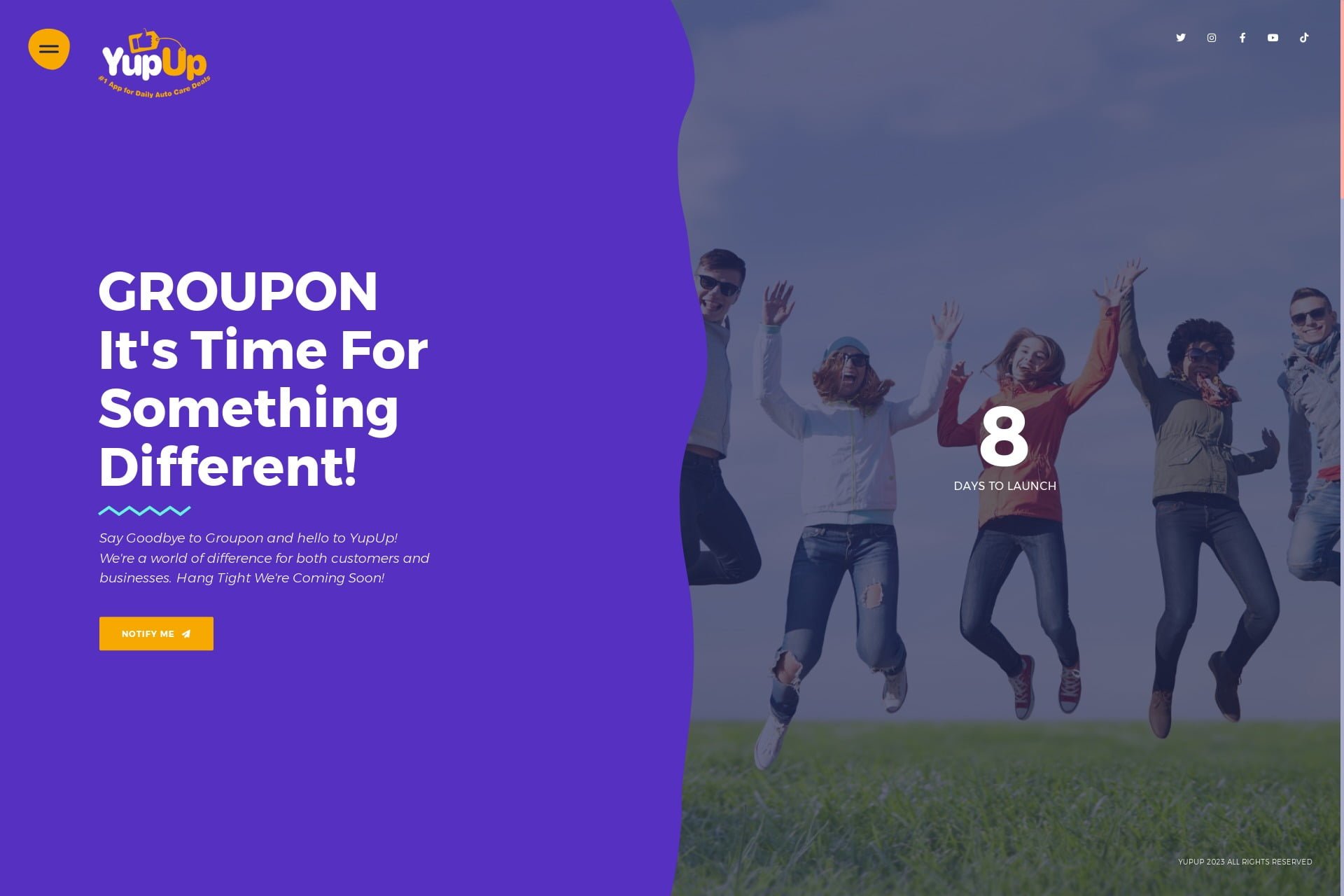Screenshot of the YupUp Website:

At the top left of the webpage, the YupUp logo is prominently displayed, featuring a playful bubble font. The word "Yup" (spelled "W-U-P") appears in white, while the word "Up" (spelled "U-P") is in yellow. Below the logo, there is some small, unreadable text. To the top right, a set of social media icons is neatly arranged.

The main body of the webpage is divided into two sections. On the left side, a large blue background dominates the space. Overlaying this background is a bold white text that reads, "Groupon, it's time for something different." Beneath that, in smaller text, it says, "Say goodbye to Groupon and hello to YupUp. We're a world difference for both customers and businesses. Hang tight, we're coming soon." Below this message, a bright yellow button invites users to "Notify me" about updates.

To the right, an image captures a group of young people, both men and women, energetically jumping in a plain grass field, their hands raised in excitement. Above this image, large white text displays the number "8," indicating the countdown to launch with the phrase "days to launch" beneath it.